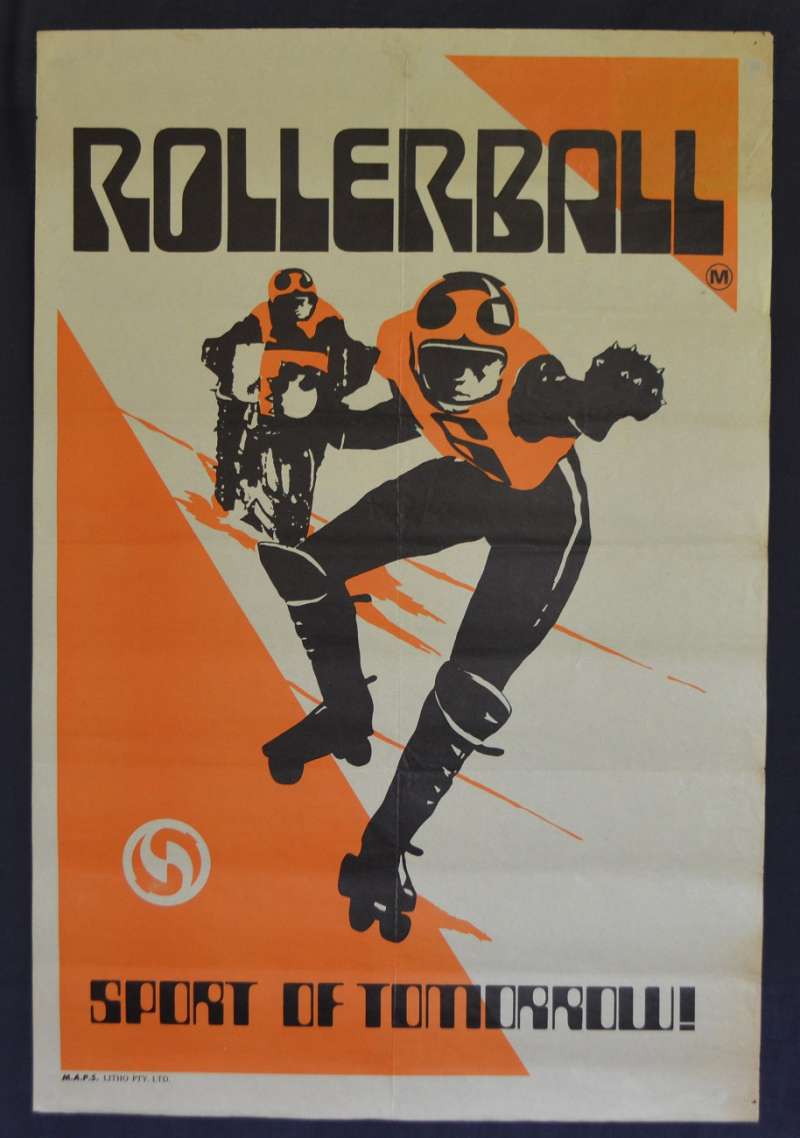The image depicts a vintage advertisement poster for "Rollerball," characterized by a vertical rectangular shape with a thick, black inner border. The background features a light brown color, overlaid with two prominent orange triangles—one large triangle emerging from the bottom left corner and a smaller one from the top right. Dominating the center of the poster is the title "Rollerball" in a bold, stylized black font reminiscent of a 1960s aesthetic.

The main focus of the poster is two figures: one on roller skates and the other on a motorcycle. Both figures are attired in striking black and orange uniforms, featuring orange helmets, black pants, and orange vests with numbers, including the visible number six. The motorcycle incorporates a matching color scheme of black and orange. Positioned beneath these dynamic figures is the tagline "Sport of Tomorrow," emphasizing the futuristic nature of this sport. The overall design and color choices create an action-packed, high-energy feel, evoking the thrilling and fast-paced essence of Rollerball.